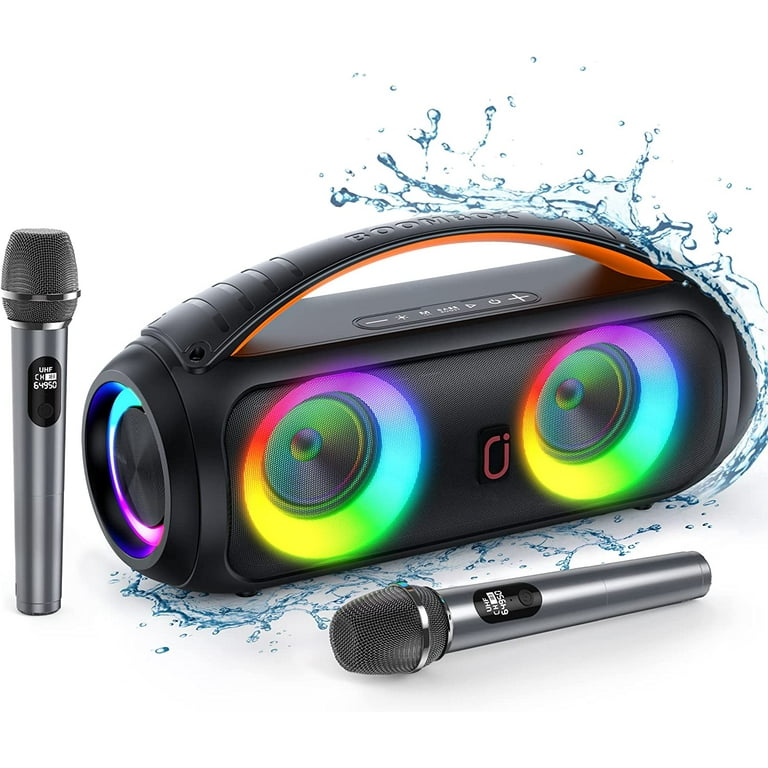This is a close-up angled view of a sleek, black karaoke machine with an old-school boom box shape, set against a white background. It features a prominent arched handle that spans the length of the device. The front of the machine displays two round speakers illuminated by neon lights in a vibrant color wheel pattern of yellow, blue, red, and purple. A small flat speaker on the left side is bordered by a thin strip of neon lights in teal, pink, and purple. Surrounding the machine is a stylized water splash graphic, indicating that it is waterproof. In front and to the left of the machine are two silver microphones with black tops—one lying horizontally and one standing vertically. The image appears digitally altered, emphasizing a modern, ad-like aesthetic with a transparent background.